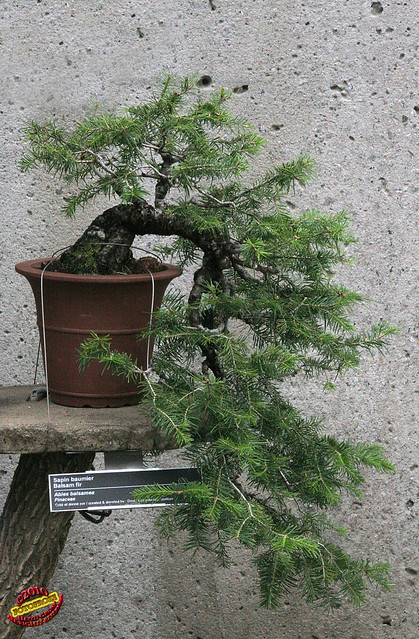This image captures a quaint scene featuring a small bonsai pine tree, specifically a balsam fir, in a brown pot. The bonsai, notable for its delicate, needle-like leaves, appears artfully trimmed with its U-shaped trunk curving downward, rather than standing straight. The pot rests on a stone shelf, supported by a tree trunk brace, affixed to a cement wall with a gray, pockmarked surface. A small black sign with white lettering, reading "sapin balmier," hangs down in front of the pot. This charming bonsai display embodies the careful pruning inherent in bonsai cultivation, set against an understated concrete backdrop.